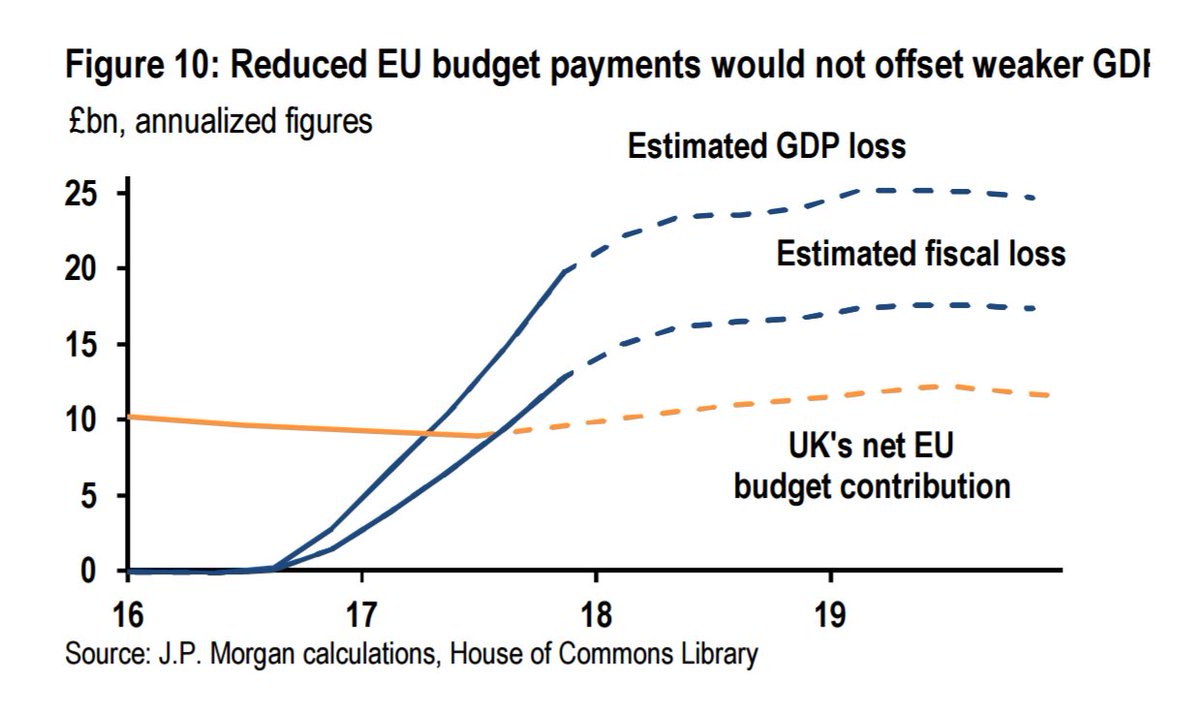This detailed horizontal rectangular image features a line graph titled "Figure 10: Reduced EU Budget Payments Would Not Offset Weaker GDI." The y-axis, labeled "Pounds in Billions, Annualized Figures," has numerical markers starting from 25 at the top and descending in intervals of 5 to 0. The x-axis includes distinct lines representing "Estimated GDP Loss," "Estimated Fiscal Loss," and "UK's Net EU Budget Contribution," with numerical markers for the years 2016 to 2019. At the very bottom, the source is cited as "JP Morgan Calculations, House of Commons Library."